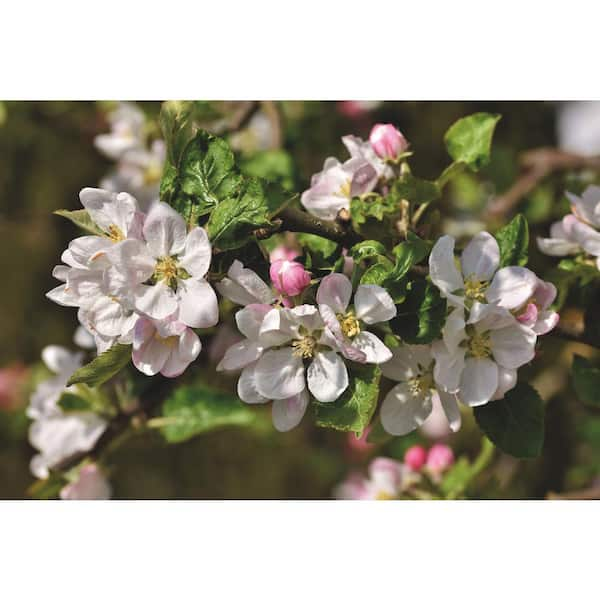The photograph captures a plant in the wild, possibly a dogwood or cherry tree, distinguished by its wooden brown branches, which appear slightly blurred due to the focus. The branches are adorned with small green leaves that have a somewhat wrinkled, spade-like shape. Interspersed among the leaves are numerous delicate flowers exhibiting a color gradient from pinkish buds to fully opened petals that are predominantly white with a subtle pink hue. Each flower has a yellow center, where tiny yellow stamens protrude, indicative of the pollination process. While some flowers are in full bloom, others remain in various stages of budding. The background of the image remains out-of-focus, emphasizing the vivid detail of the plant's floral and foliar characteristics.